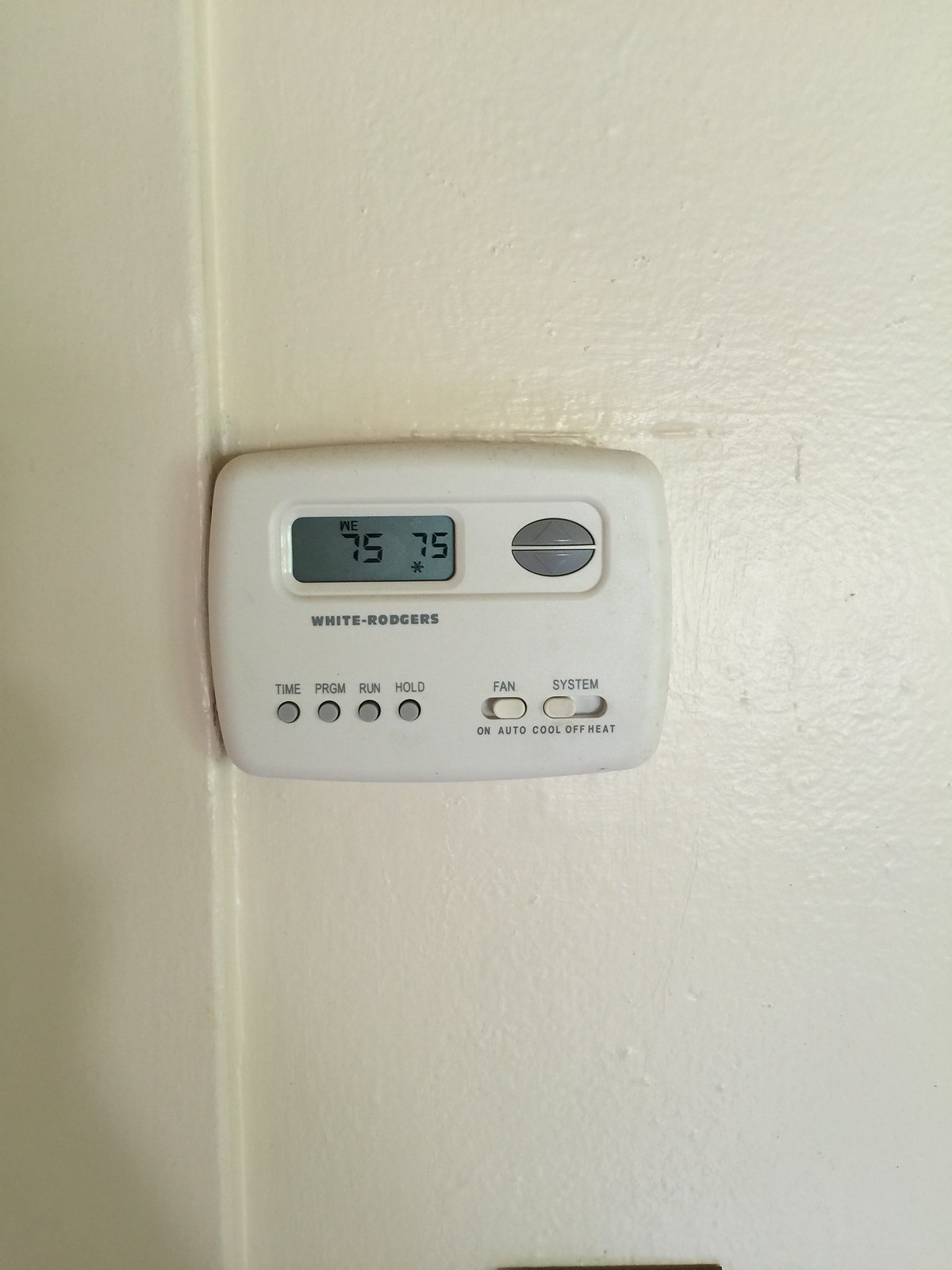The photograph depicts a rectangular thermostat centrally placed within the rectangular frame of the image, where the height is half the length of the width. The thermostat, made of light gray plastic, features a prominent rectangular indent near its top. The indent itself has rounded corners and edges, creating a soft, recessed rectangular area.

On the right side of this indent, there are two semi-circular buttons arranged to form a complete circle. The upper button has an upward-pointing arrow, while the lower button has a downward-pointing arrow, indicating temperature adjustments.

To the left within the indent, an LED screen displays information digitally. The screen, also gray, shows the current setting: "WE75-75". Beneath this indented area, white text in all capital letters spells out "WHITE-RODGERS."

In the bottom left corner of the thermostat, four round gray buttons are labeled respectively as TIME, PRGM, RUN, and HOLD. These buttons suggest functionalities associated with scheduling and temperature control.

On the opposite, bottom right corner, two sliding switches allow for further customization of the thermostat's settings. One switch toggles the FAN between ON and AUTO, while the other controls the SYSTEM with options such as COOL, OFF, and HEAT.